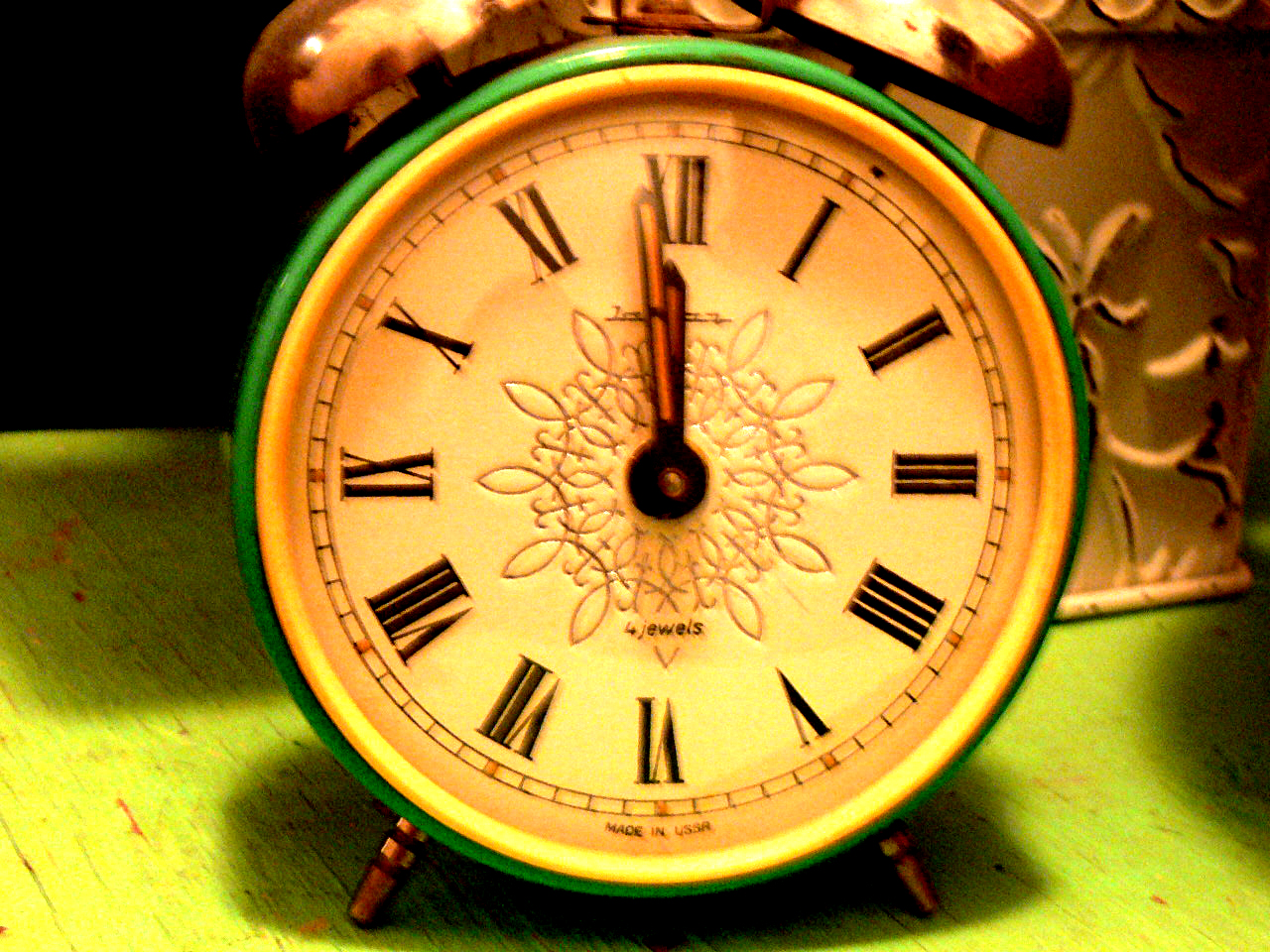An intricately designed old-fashioned alarm clock takes center stage on an end table with distinctive characteristics. The alarm clock boasts a jewel-toned green casing and is of the classic variety, featuring twin copper bells with a bell ringer in between. The clock stands on short copper legs. Its round face showcases black Roman numerals, with black hands accented in reddish tones, pointing just about to the noon hour. The center of the clock face is adorned with an elaborate mandala pattern made up of curly cues, and beneath it lies the brand name, hinting at 'four jewels' in its design.

The end table supporting this vintage timepiece is painted in a vivid lime green, with sporadic red streaks that seem to be the result of years of wear, adding to its charm. In the background, a textured white lamp with a distressed floral or ivy-stamped metal design completes the scene, imbuing the setting with a nostalgic vibe.